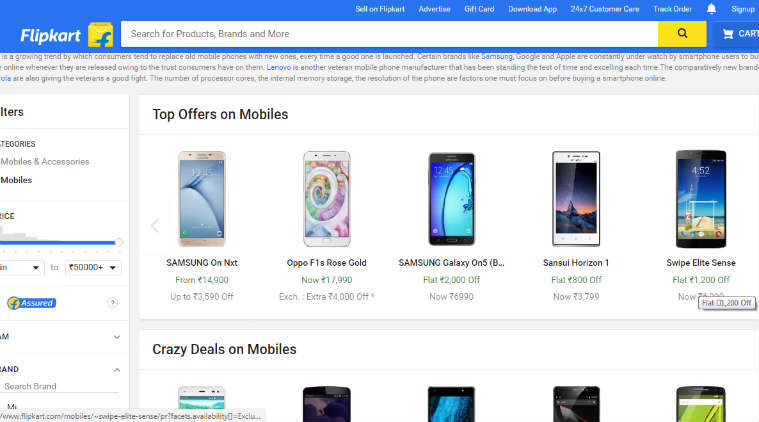The image depicts a website displayed on a computer screen, primarily showcasing mobile phones available for sale on Flipkart. At the very top of the webpage, a prominent bright blue ad banner features the Flipkart logo, characterized by a partially cut-off blue 'F' blended into a yellow field, accompanied by a search bar. The overall design of the website is minimalistic, with a white background contrasted by sections of blue and black text accents.

Beneath the ad banner, the webpage highlights top offers on mobile phones. Five distinct mobile phones occupy the upper section of the screen, displayed neatly in a row. Further down, the page transitions into a segment labeled "Crazy Deals on Mobiles," though the text is partially visible. In this section, the upper portion of five flip phones is evident.

In the upper right-hand corner of the screen lies a vibrant yellow search button, completing the interface and inviting users to search for specific items. The clean layout and strategic use of color make the website user-friendly and visually engaging, focusing the viewer's attention on the diverse mobile phone offers.